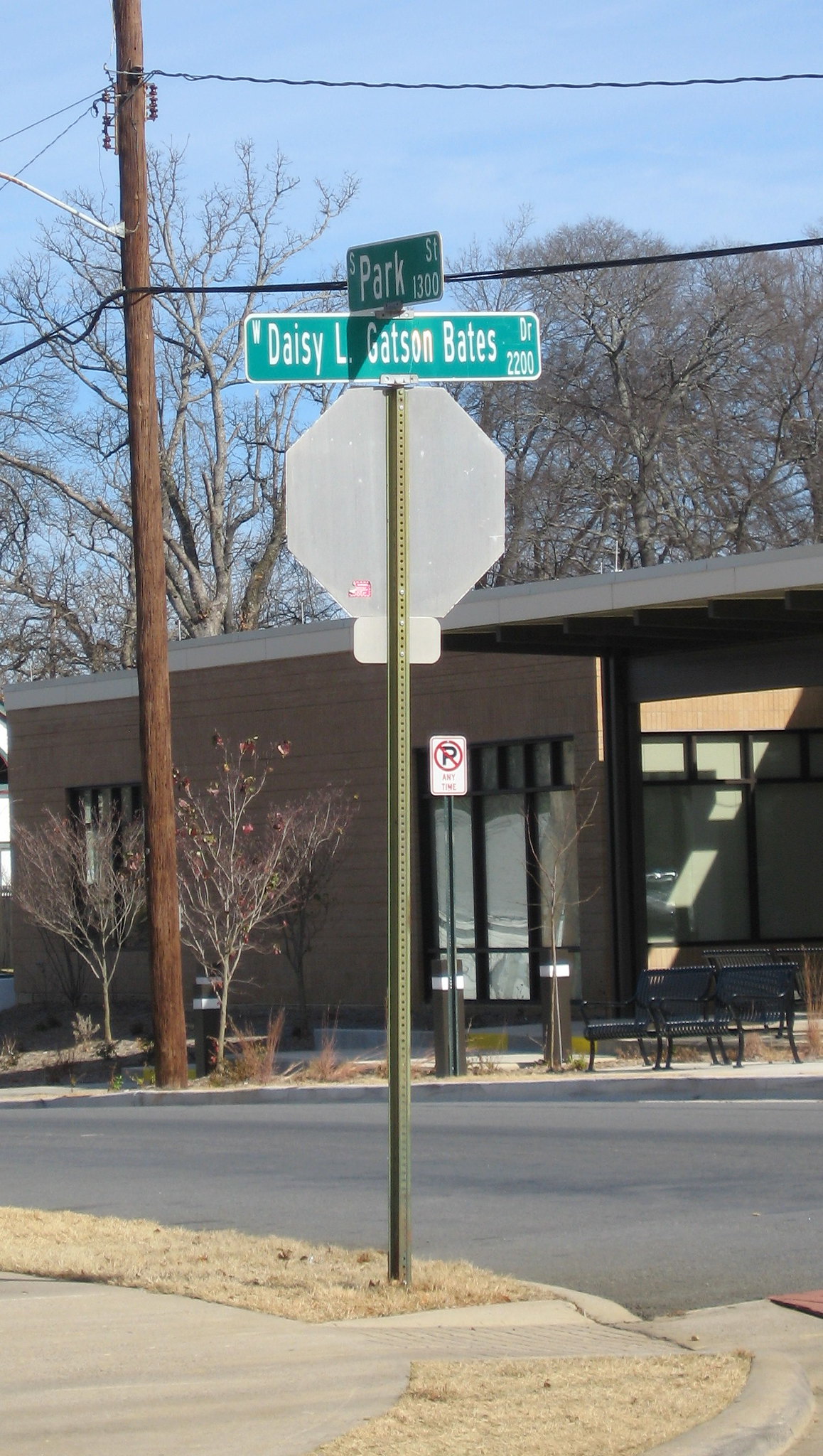In this urban scene, the focus is on a street corner featuring a prominent street sign. The corner includes a curb and a sidewalk, with the street sign displaying two green panels at the top. The right-facing sign reads "Daisy L. Gatson Bates Drive 2200," while the front-facing sign indicates "South Park 1300 Street." Across the street to the right, a telephone pole with an attached electrical wire stands in front of a low, brick building. This brown building is characterized by its long front windows. In front of the building, there is a metal bench, and nearby, a white 'No Parking' sign with a red circle and a crossed-out black 'P' is clearly visible.